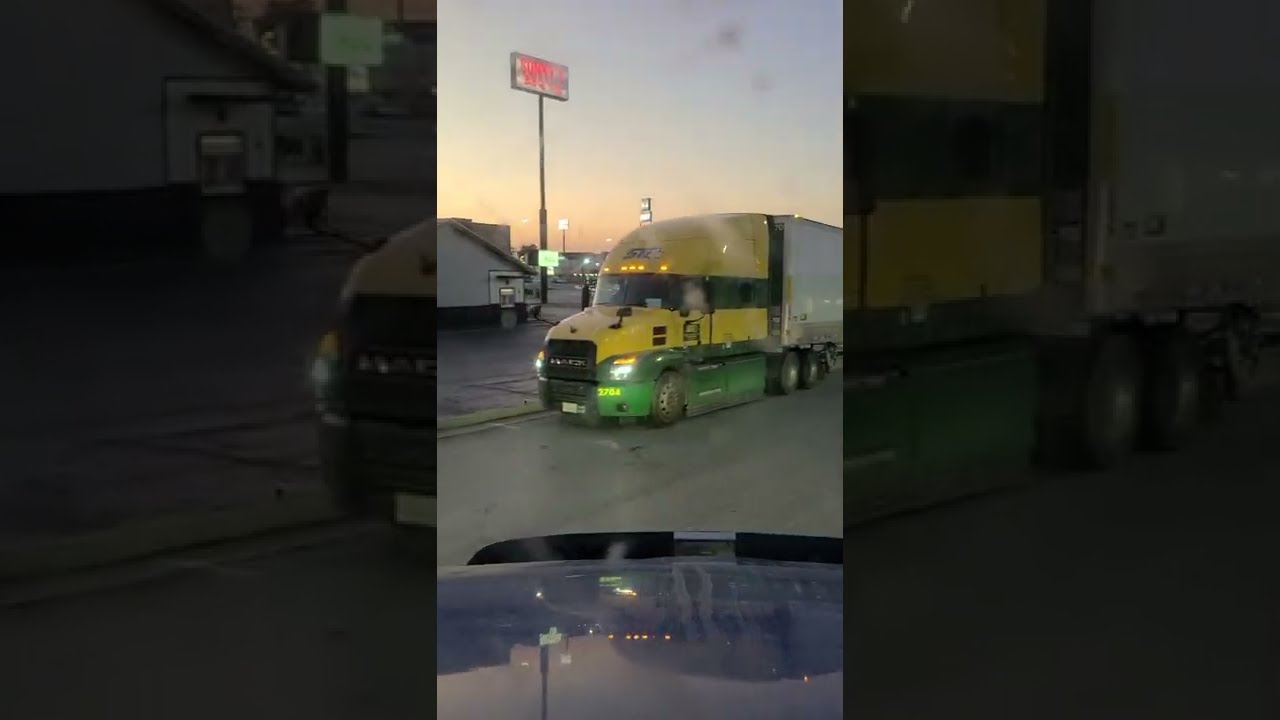The photograph features a yellow and green semi-truck hauling a large white cargo box, captured facing three-quarters to the left. The truck spans the middle third of the image horizontally, extending from bottom to top. The photograph is viewed from the hood of another blue truck in the foreground. The semi-truck has large front windows and its headlights are on, suggesting it is nearing dusk. In the background, there's a white building on the left side and a tall black pole with a red and white business sign atop, though the text is unreadable. The sky displays a gradient from blue at the top to orange near the horizon, indicating either sunrise or sunset. Additionally, the photograph overlay includes zoomed-in and darkened versions of the same image on its left and right thirds, focusing on the area with the semi-truck and its surroundings.